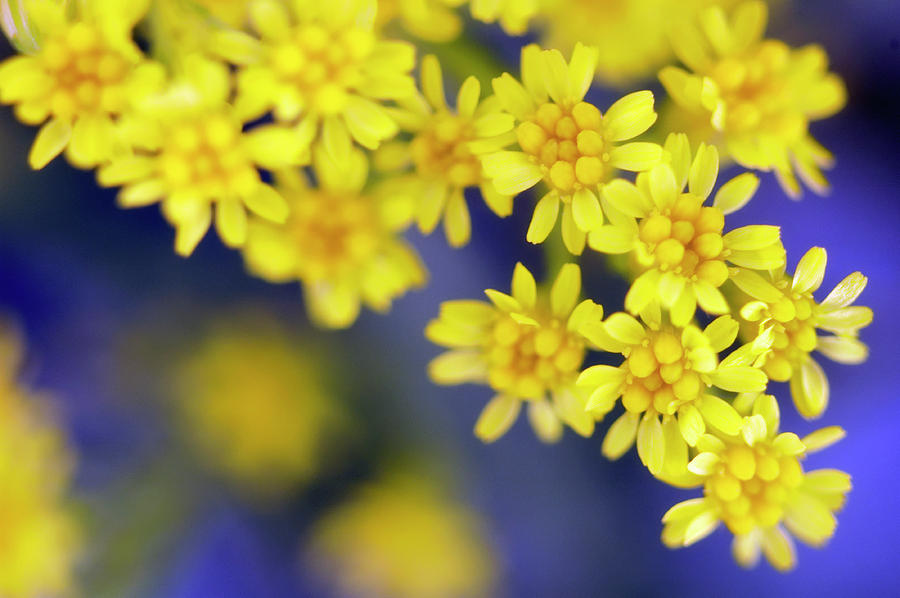This high-quality close-up photograph captures a vibrant cluster of bright yellow Goldenrod flowers, emphasizing their intricate details and vivid coloring. The small, elongated petals surround bulbous yellow centers, creating dense floral sprays descending at an angle from the top of the image towards the bottom right. The cobalt blue backdrop, coupled with patches of sunlight, enhances the flowers' bright school bus yellow hue, making them appear especially vibrant. The background is subtly blurred, showcasing additional clusters of yellow flowers and deep purple patches, further highlighting the foreground's intricate floral details. This perennial wildflower, belonging to the aster family, is often found growing along roadsides.